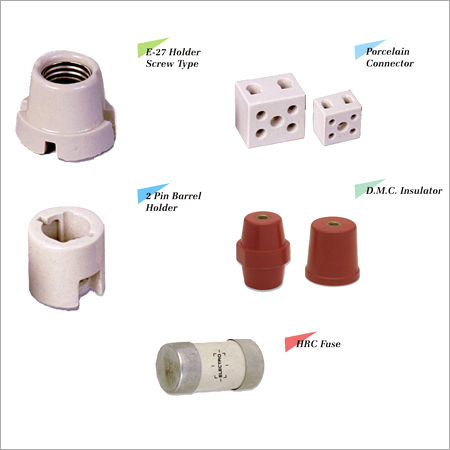The image is a square photograph featuring various electrical components set against a solid white background, each outlined by a thin black border. In the upper left-hand corner, there is a cylindrical object with a white exterior and a silver interior, labeled "E-27 holder" and "screw type" in small black text. To the right, occupying the upper right-hand corner, are two porcelain connectors that resemble dice; the larger one is on the left, and both are tagged as "porcelain connector" in small print. Below that, towards the middle left of the image, is another completely white cylindrical object marked as a "two pin barrel holder." To its right are two red, cylindrical items named "DMC insulator," featuring holes at their tops. At the bottom center of the image, a small vial-like object, tilted on its side, carries the label "HRC fuse." All these components, five in total, represent different types of electrical hardware.